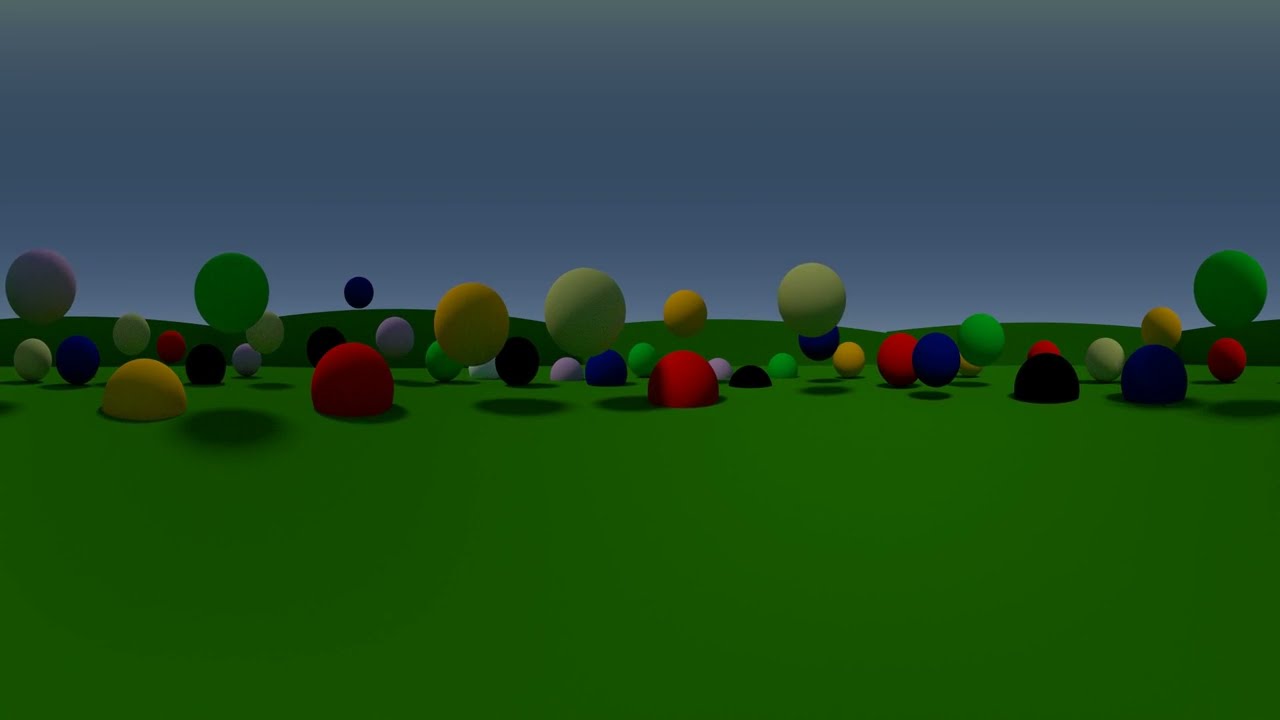This image is a basic 3D computer-generated landscape showcasing a grassy field with undulating hills in the background. The scene features a multitude of colorful spheres in various states of elevation; some are floating just above the grassy surface while others are partially embedded within it or resting atop. The grass itself is a uniformly flat green, devoid of intricate textures. The sky above transitions from a lighter hue near the horizon to a darker blue towards the top, evoking a sense of either sunrise or sunset. The spheres vary in color, including shades of yellow, red, blue, green, black, and white, and their sizes differ slightly, with some spheres being approximately twice as large as others.